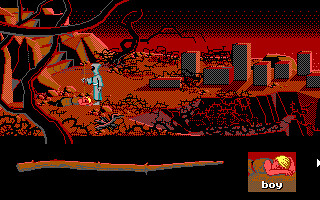The image captures an intense scene from a video game, set in a post-apocalyptic wasteland. The sky is a haunting blend of red and black, casting an ominous hue over the desert-like landscape below, which is tinged in orange and dotted with eerie black and red branches. A figure in a hazmat suit, resembling a grim reaper, stands prominently in the middle. The figure is donned in an off-white robe with a black mask-like object on their face. Below them lies a dead body with a reddish skin tone, wearing an orange outfit. Scattered around the corpse are skulls in black and orange. On one side of the image, a menacing red pit is overgrown with black and red vines. The background features gray block-like structures, lending an industrial decay to the scene. In the foreground, there is a red, olive, and yellow-faced image of a person lying on the ground with the word "boy" in white font below it. The bottom of the image is dominated by a large, orangey-tan tree branch, adding to the desolate and foreboding atmosphere.